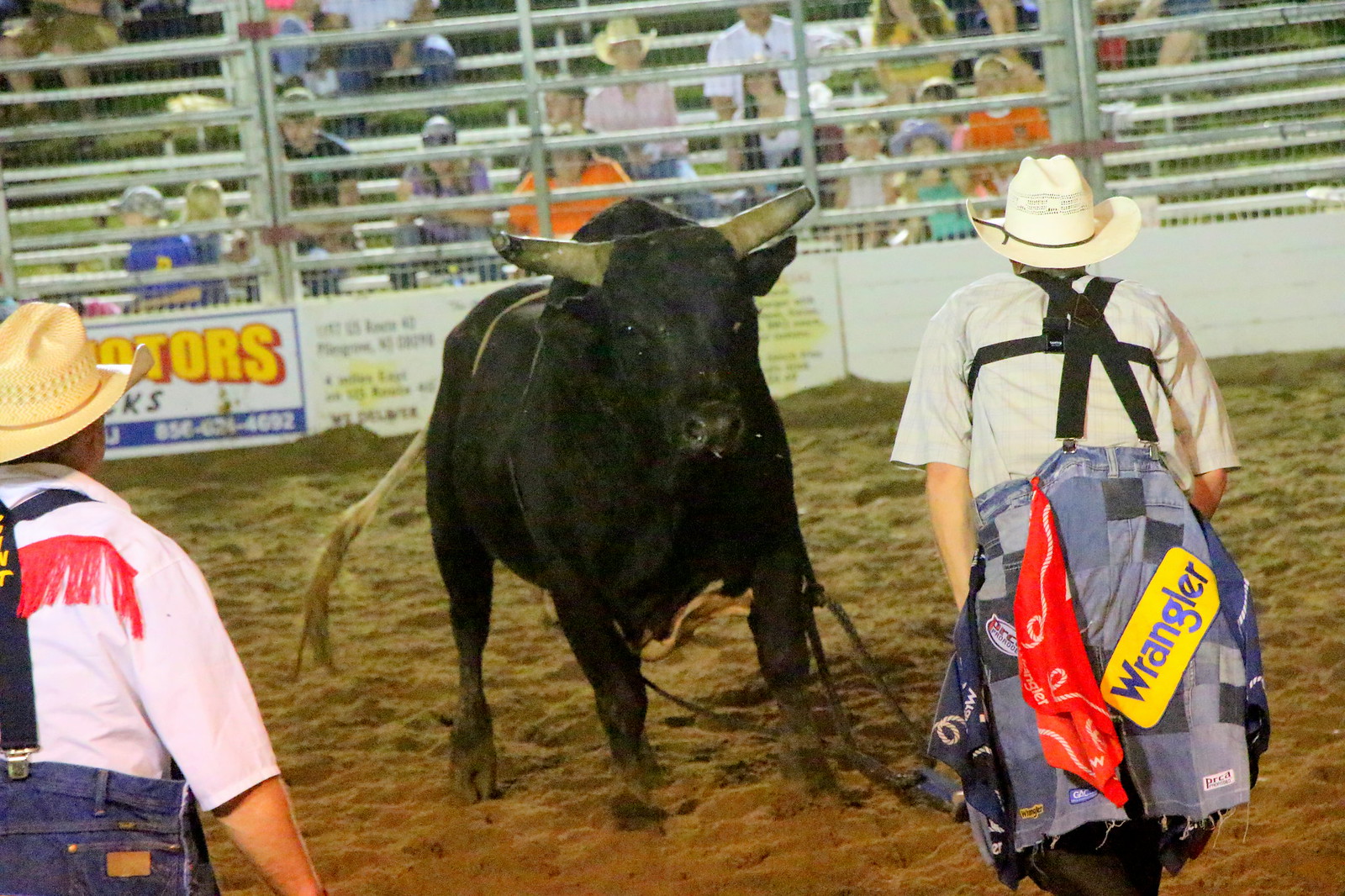In the center of a dusty rodeo arena, a large black bull with filed-down horns and a white tail stands, poised and seemingly staring at a man on its left. This man is dressed in a white shirt with a white cowboy hat, and suspenders holding up a blue jacket tied around his waist, the word "Wrangler" emblazoned in big blue letters against a yellow background. On the right, another man, dressed in a similar outfit with a yellow cowboy hat, white shirt, and suspenders attached to his blue jeans, faces the bull. Both of these men, who appear to be rodeo clowns, are intently focused on the bull, which seems prepared to charge. Surrounding the arena, behind a sturdy wire fence and additional metal gates designed to keep the bulls enclosed, spectators fill the bleachers. Various advertisements, including one with the word "motors," are visible along the fence line at the bottom edge of the bleachers, adding a colorful backdrop to the tense scene unfolding in the center.